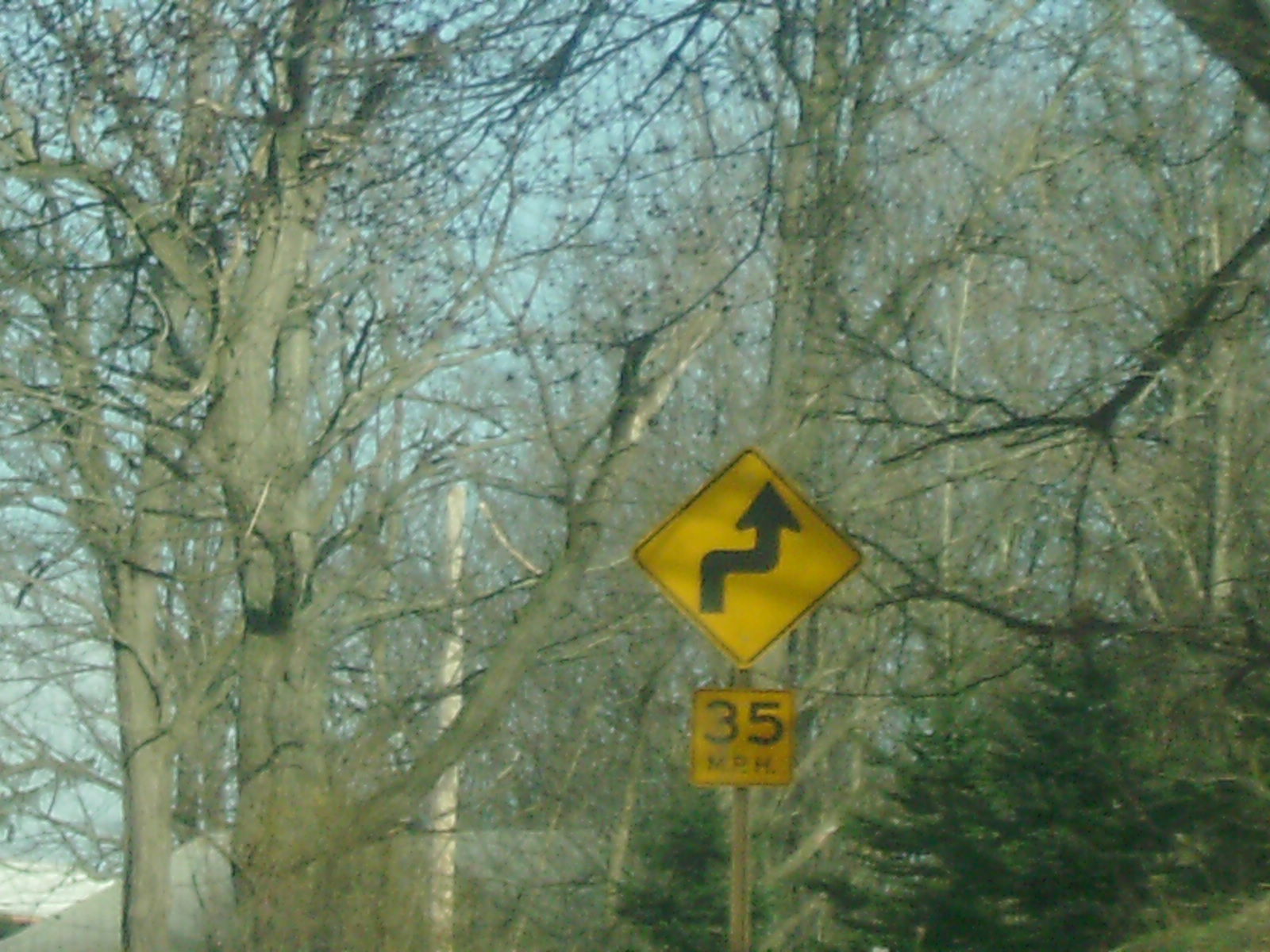The image features a yellow traffic sign, diamond-shaped like a rotated square. The sign displays a black, squiggly arrow pointing upwards and to the right, ending in a triangle, indicating a winding road ahead. Below this, there's a smaller yellow square sign with "35 MPH" in bold black text, suggesting the speed limit. Both signs are mounted on a gray pole.

In the left and right foreground, large, dead trees dominate, showcasing thick branches adorned with numerous stubby offshoots. To the right of the sign, there are also about four smaller, healthy trees, providing a contrast to the otherwise desolate landscape.

In the distant background, a striking dead tree with a pale, almost white trunk stands out, reminiscent of the iconic Tree of Gondor from fantasy lore. The scene is set against a backdrop of clear blue skies, adding a touch of serenity to the otherwise stark and haunting environment.